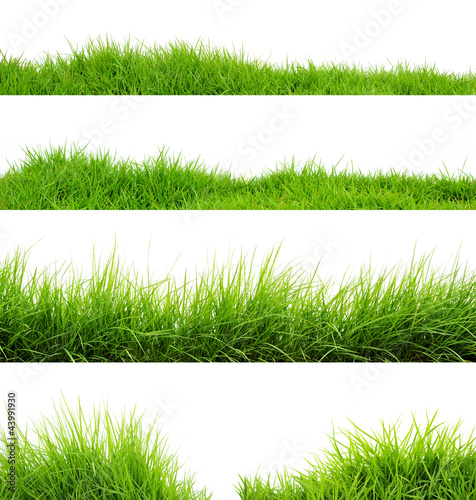The image is a vertical, rectangular panel divided into four rows, each showcasing various stages of lush green grasses against a pristine white background. The top two rows feature very fresh, short green sod grasses, vividly capturing their newly grown essence. The grasses in the left column of these rows are slightly taller than those on the right. In the third row, the grass appears much taller and seems to be swaying gently as if blown by the wind, with a white sky visible behind it. The bottom row presents another view of tall grasses, but here, the grass is noticeably parted, creating a gap in the middle, while remaining thick and tall on both sides. The word "Adobe Stock" is diagonally printed across the whole image, and in the bottom left corner, it says "Adobe Stock" with a vertical line separating it from the code "43991930".